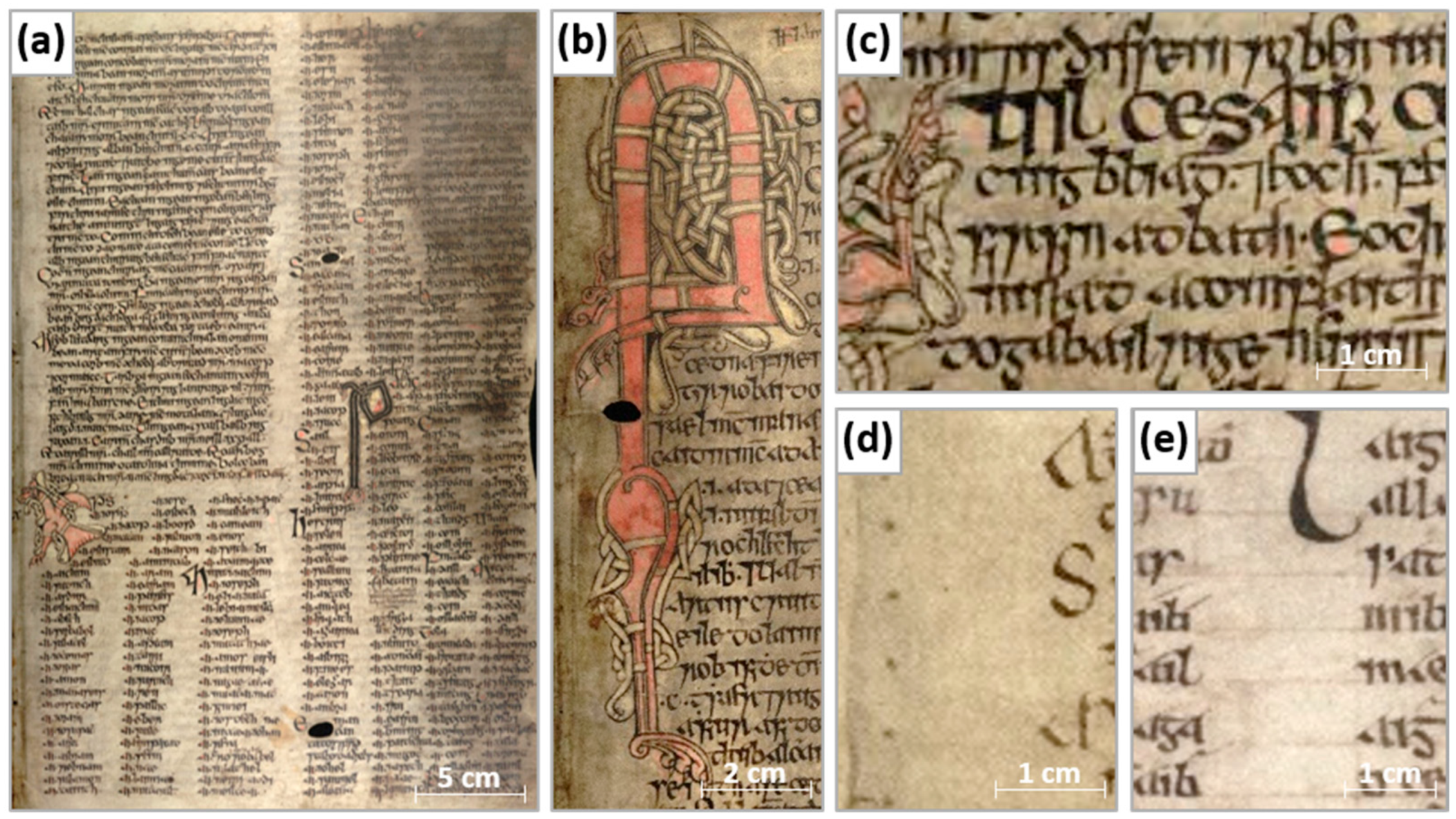This image is composed of five panels labeled A, B, C, D, and E, each depicting a section of a very old and aged book. The panels correspond to measured widths, with panel A being 5 cm, panel B 2 cm, and panels C, D, and E each 1 cm in width. The pages display text in an undecipherable, almost medieval script, resembling an ornate, possibly ancient language. The pages are visibly worn, with dirt and age marks, though the black ink remains sharp and clear, while the reds are fading. Panels B and C feature red ornate designs, adding to the historical and possibly Celtic or Elvish appearance of the text. The overall impression is that of an ancient manuscript, potentially hundreds or thousands of years old, showcasing intricate and mysterious writing.